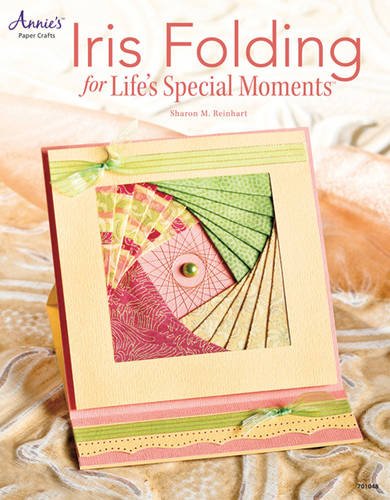The image is a vertically oriented advertisement for a product designed for storing pictures or other cherished memories. Dominating the center is a slightly tilted, square picture frame with a light yellow border and a green ribbon draped across the top. Inside the frame, various fabric samples are arranged, including a green spotted fabric, a yellow striped fabric, a purple striped fabric, and a colorful blend of green, purple, and yellow blotches. Central to this design is a gold ball resembling a bearing, encircled by a spider-web-like pattern. The background features an orange and white swirling surface that appears to be a decorative sheet or tablecloth. In the top left corner, the brand "Annie's Paper Crafts" is inscribed in purple cursive. Prominently across the top, the bold red text reads "Iris Folding for Life's Special Memories," with smaller text below attributing the design to Sharon M. Reinhart. The overall effect is a vibrant and detailed display, suggesting a product related to photo albums or crafting.